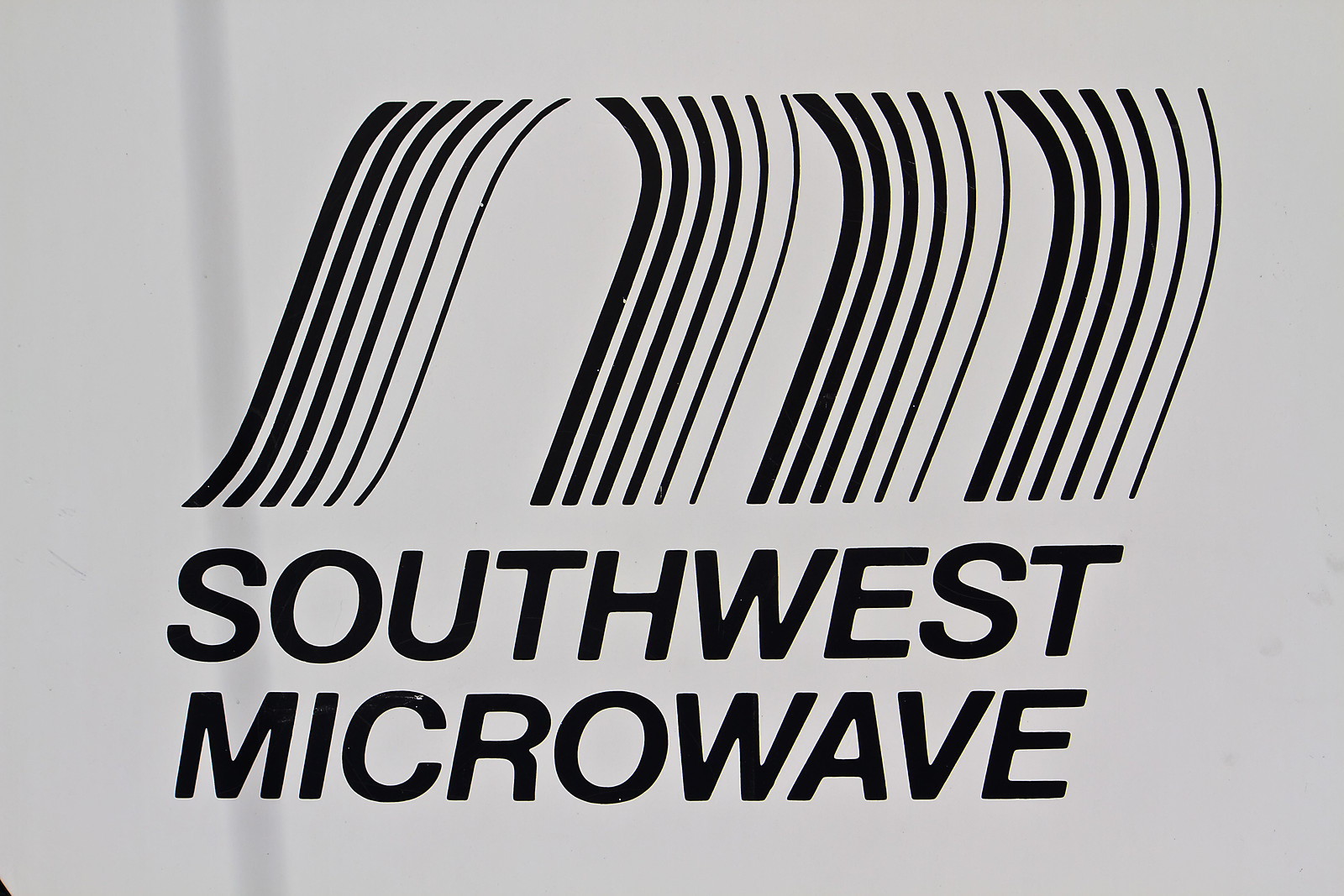The image features the text "Southwest Microwave" prominently displayed in large, capitalized, italic, and sans-serif black letters on a white background. Above this text, there is an abstract logo consisting of several thick, black lines forming an incomplete or stylized letter "M" or "N" shape, with the tops of the lines curving or cut off, creating a layered, swirl-like effect. The design and the text are both in striking contrast against the plain white background, with a slight shadow visible to the left of the text, particularly near the "S" and "M" of "Southwest Microwave." The overall aesthetic is minimalistic, giving the impression of a company logo or sign.